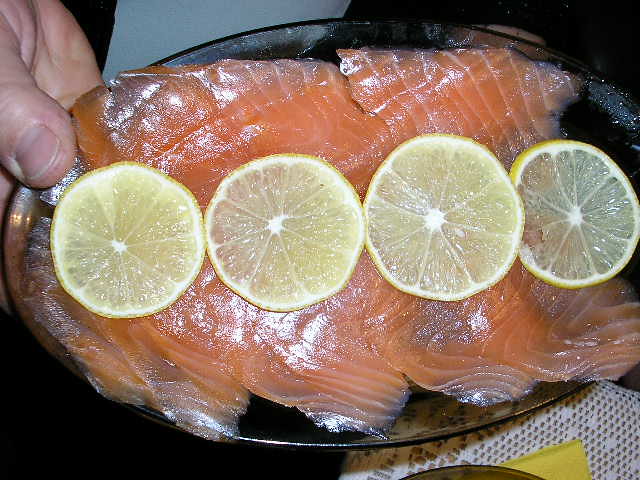This is a color photograph taken with flash, showcasing a circular glass dish with a gold rim, filled with thinly sliced raw salmon, identifiable by its distinctive orange, slightly translucent flesh at the edges. The salmon slices cover the majority of the dish and are accompanied by four thinly sliced lemon rounds neatly placed across the center of the fish. In the upper left corner of the image, a Caucasian person's thumb and part of their hand are visible as they hold the plate. The background is primarily filled with shadow, though a white lace tablecloth and a small, indistinct yellow piece of paper can be seen in the bottom right corner. The severe reflection of the flash creates a bright glare on both the fish and lemons, enhancing the details and the texture of the raw salmon.